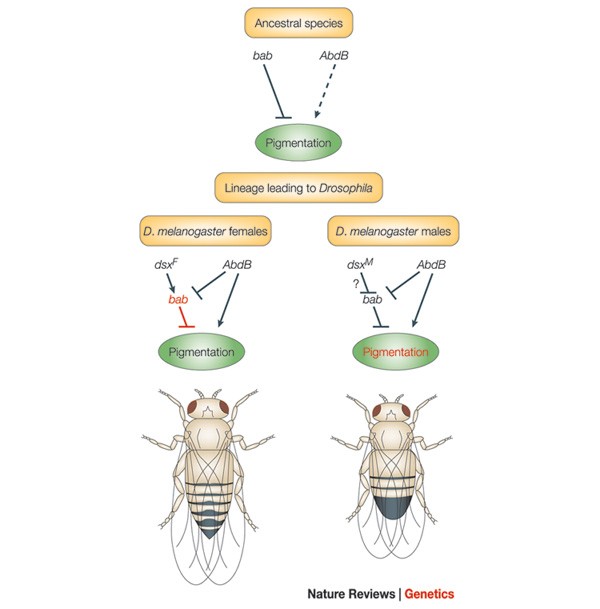This vertical image, lacking an external border, serves as an educational graphic explaining the genetic differentiation of a specific bug species, likely Drosophila, based on their pigmentation traits. At the very top, the title "Ancestral Species" is followed by a diagram that traces genetic elements labeled as BAB and ABDB, with arrows pointing to an oval marked "Pigmentation." Below this is a lozenge-shaped box labeled "Lineage Leading to Drosophila." The diagram further bifurcates into two sections: on the left, "D. melanogaster females," depicting a larger bug with big eyes, translucent wings, six legs, antennae, and a striped body; and on the right, "D. melanogaster males," showing a slightly smaller bug with similar anatomical features. The distinctions between the male and female bugs, particularly in size and pigmentation, are highlighted. At the bottom, the text reads "Nature Reviews" in black, separated by a vertical line, followed by "Genetics" in red. This detailed visual guide visually communicates the genetic lineage and the differences between male and female Drosophila.